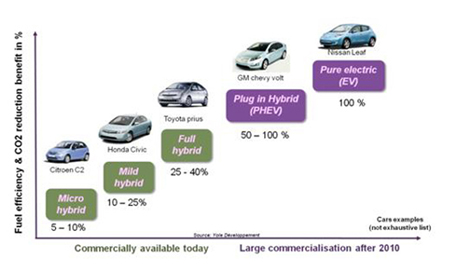This is a detailed graph illustrating the fuel efficiency and CO2 reduction benefits of various types of vehicles, measured in percentages on the y-axis. The x-axis is divided into two sections: "Commercially Available Today" (labeled in green) and "Large Commercialization After 2010" (labeled in purple). The trend of the graph is upwards, reminiscent of a y = x graph.

On the left side, under "Commercially Available Today," three types of hybrids are depicted. Starting from the bottom, there is a micro-hybrid with fuel efficiency and CO2 reduction benefits ranging from 5% to 10%, exemplified by a Citroen C2. Higher up, with benefits ranging from 10% to 25%, is the mild hybrid, represented by a Honda Civic. At the top of this section, showing a 25% to 40% improvement, is the full hybrid, illustrated by a Toyota Prius.

On the right side, under "Large Commercialization After 2010," two types of vehicles are shown. The plug-in hybrid electric vehicle (PHEV) demonstrates a 50% to 100% benefit and is embodied by a GM Chevy Volt. Above it, displaying a 100% benefit, is the pure electric vehicle (EV), represented by a Nissan Leaf.

Each vehicle type is accompanied by a label showing its category, and the graph highlights the increasing trend in fuel efficiency and CO2 reduction benefits as you move from left to right and bottom to top.